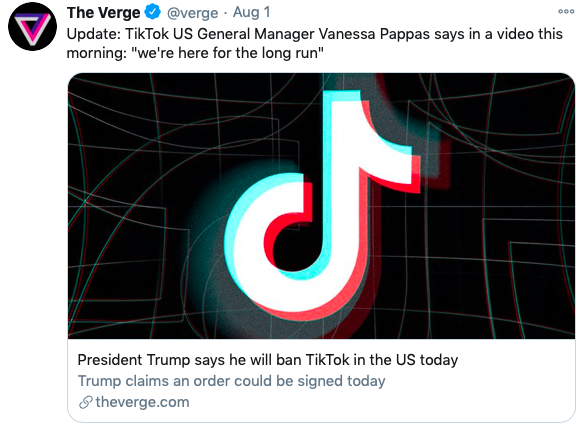Here is the cleaned-up and detailed caption for the described image:

---

The image is a screenshot of a tweet posted by The Verge, identifiable by their username and logo—a black circle with a pink and lavender triangle—visible in the upper-left corner. The tweet, dated August 1st, includes an update from TikTok's US General Manager, Vanessa Pappas, stating via a video that morning, "We're here for the long run." Below this text, the news story's image features a simple black background with the TikTok logo, which resembles a musical note in white, outlined with light blue and light red accents. The headline below the image reads, "President Trump says he will ban TikTok in the US today," followed by the subtext, "Trump claims an order could be signed today," and the source, "theverge.com."

---